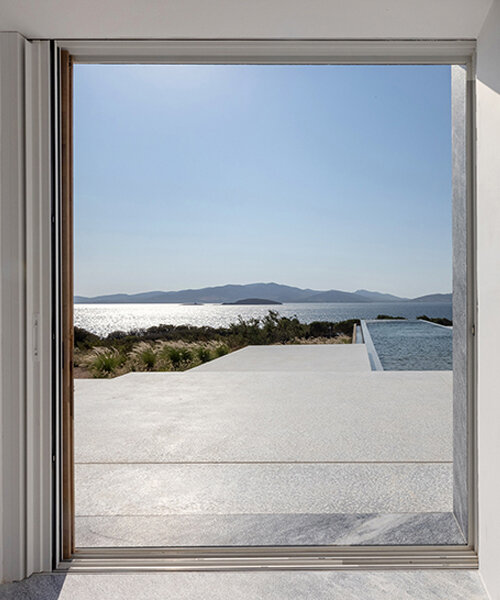The photograph captures an outdoor scene viewed through a vertically oriented, open window with a grayish stone frame, possibly made of concrete, granite, or marble. The window itself is clean and white, devoid of any glass, creating an unobstructed view. Right outside the window, there is a grayish white concrete patio or walkway with different levels, featuring some steps that lead down to a sandy area interspersed with grasses, shrubs, and nondescript external structures.

Beyond this immediate foreground lies a rectangular pool, followed by a lake that is expansive enough to resemble an ocean. The scene continues with clusters of bushes near the water's edge and small, distant mountains that add depth to the background. The photograph is taken during the daytime under a clear blue sky, showcasing the serene natural landscape in its full splendor.